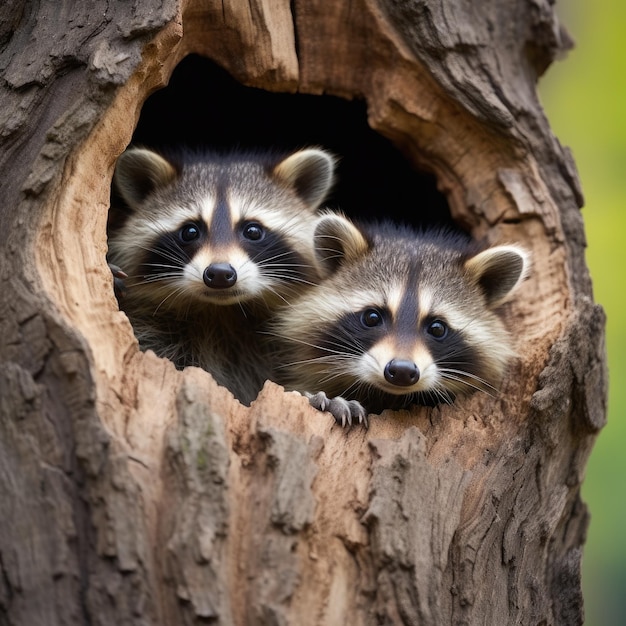This is a detailed color photo of two small baby raccoons peering out from a hole in a large tree trunk. The focal point of the image is the unique carved-out hole in the thick brown bark of the tree, which has evident growth rings. The raccoons, likely young given their size, are nestled within this dark, cavernous hole. One raccoon has its paw resting on the edge of the tree stump, while the other stares directly out. Both have distinctive black patches of fur around their beady black eyes, with light fur extending above their eyes that resemble eyebrows. The fur on top of their heads is a blend of dark and light hairs, and their ears appear with light outer rings and darker inner sections. A stripe of brown runs down the center of their cute, flat noses. The background is out of focus, with a wash of green foliage, emphasizing the clarity of the raccoons and the tree. This AI-generated image captures a very clean and detailed scene of these adorable creatures in their natural, wooded habitat.